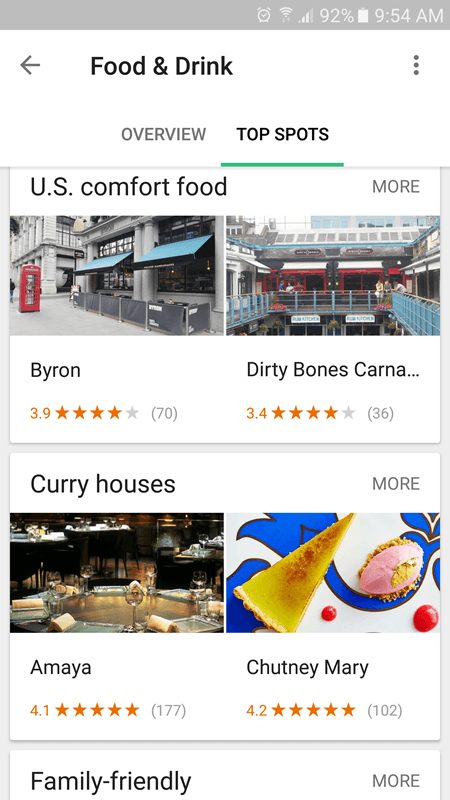This is a screen capture from a cell phone displaying a food and drink website with a white background in a vertical, rectangular format. The top of the screen features a black header that reads "Food and Drink," followed by "Overview." Below that, "Top Spots" is highlighted with a green bar, accompanied by the text "U.S. Comfort Food." The upper section of the screen showcases two photographs depicting the exteriors of food establishments. The left photograph features a place called "Byron," rated 3.9 stars, while the right photograph displays "Dirty Bones Karna," rated 3.4 stars. 

The lower section labeled "Curry Houses" includes two additional photographs. The left image appears to show a tabletop setting, representing "Amaya," and the right image features a slice of pie with a small scoop of what looks like ice cream, representing "Kutney Mary." At the bottom of the screen, the caption "Family Friendly" is displayed in black letters.